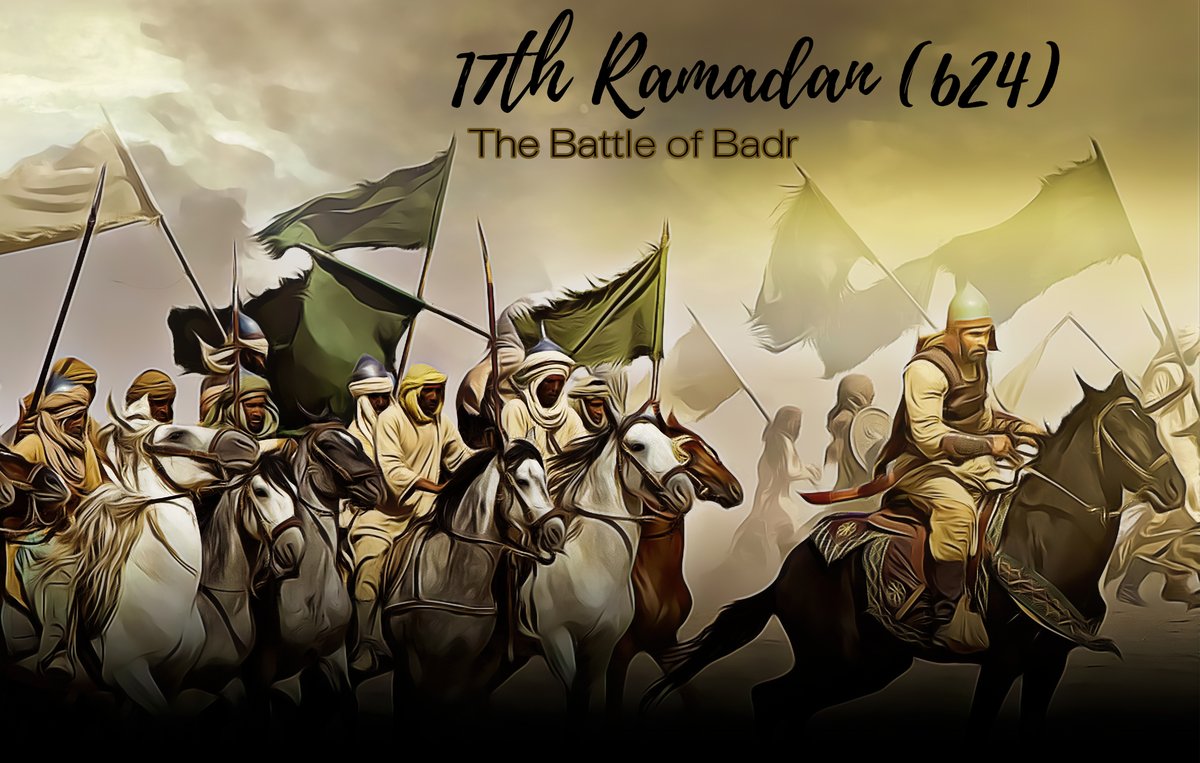The image is a computer-generated, artistic illustration set in a landscape format, depicting the Battle of Badr, which took place on the 17th of Ramadan in the year 624. The top of the image features text in bold, black script and sans serif font, which reads "17th Ramadan, 624" with "the Battle of Badr" below it. This text is set against a backdrop of dark, smoky clouds, creating a dramatic atmosphere.

In the foreground, a variety of men are seen riding different colored horses, including brown, white, gray, and black. These men are clad in Arabian-style robes, turbans, and some wear pointy helmets and protective vests. They carry flags, predominantly in shades of green, signifying their allegiance, and some also wield spears, indicating they are ready for battle.

The background is hazy, with light filtering through blurred clouds, adding to the swirly and slightly abstract artistic style of the illustration. The men, despite wearing culturally appropriate attire and armor, are depicted with a determined look, all focused in the same direction as they advance on horseback, suggestive of their united purpose in the historical battle.